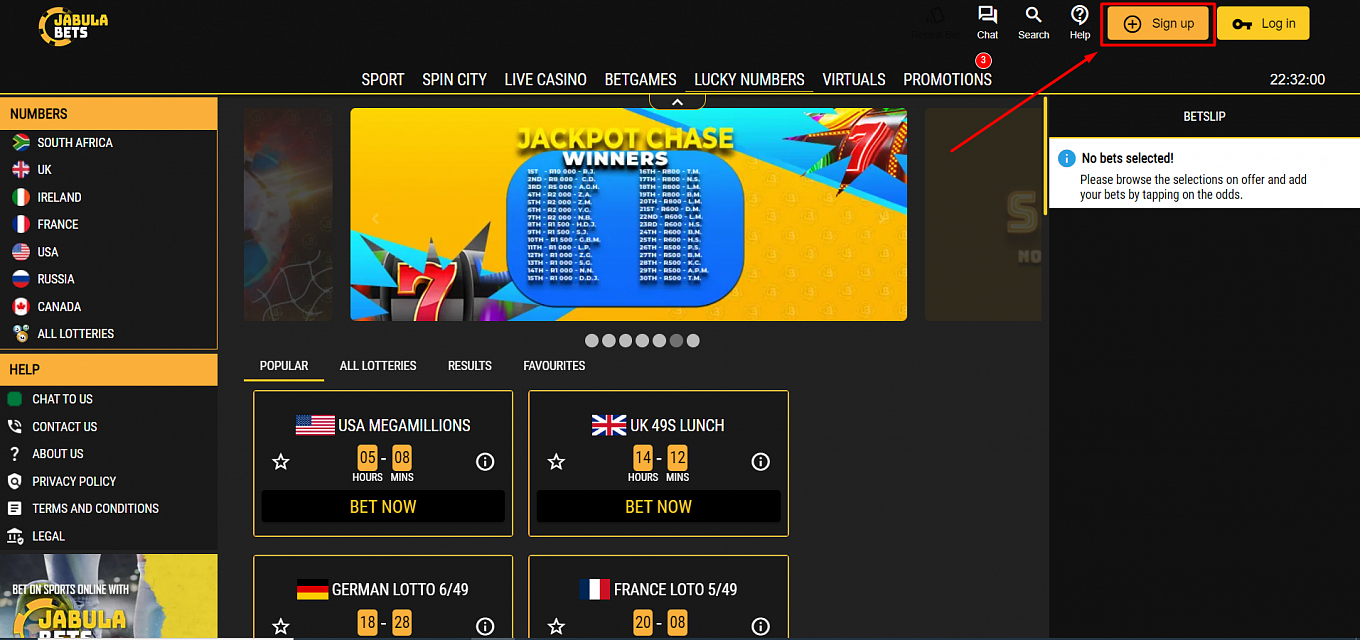**Detailed Caption:**

This is a screenshot of the Jabula Bets betting website. The interface primarily features a black background highlighting the brand name "Jabula Bets" in the top left corner. The navigation menu stretches across the top of the page, offering various options: Sport, Spin City, Live Casino, Bet Games, Lucky Numbers, Virtual, and Promotions. Above the Promotions tab, a red circle with the number 3 indicates the count of promotional offers.

The left-hand column, distinguished by an orange background, is dedicated to Numbers. Below this section, the website displays icons of various flags representing different countries, including South Africa, the UK, Ireland, France, the USA, Russia, and Canada. Beneath these flags is a link labeled "All Lotteries." Further down, a Help tab offers assistance with options like Chat to Us, About Us, and Terms and Conditions.

To the right of this column, a rectangular image with a predominantly orange background grabs attention. This graphic features red sevens, akin to lottery symbols, and is titled "Jackpot Chase Winners." It lists the prizes from 1st through 30th place, along with the initials of the winners next to the respective prize amounts.

Under this visual, the Popular tab is underlined, emphasizing its active state. Adjacent options include All Lotteries, Results, and Favorites. Beneath this section, flags corresponding to different countries are displayed alongside relevant lottery information. For example, the American flag accompanies the USA Mega Millions, which notes a betting closing time of 5 hours and 8 minutes, along with a "bet now" call to action. Similar details are available for the UK and other regions.

On the page's right side, a Bet Slip section states "No Bets Selected." It prompts users to browse available selections and add their bets by tapping on the odds.